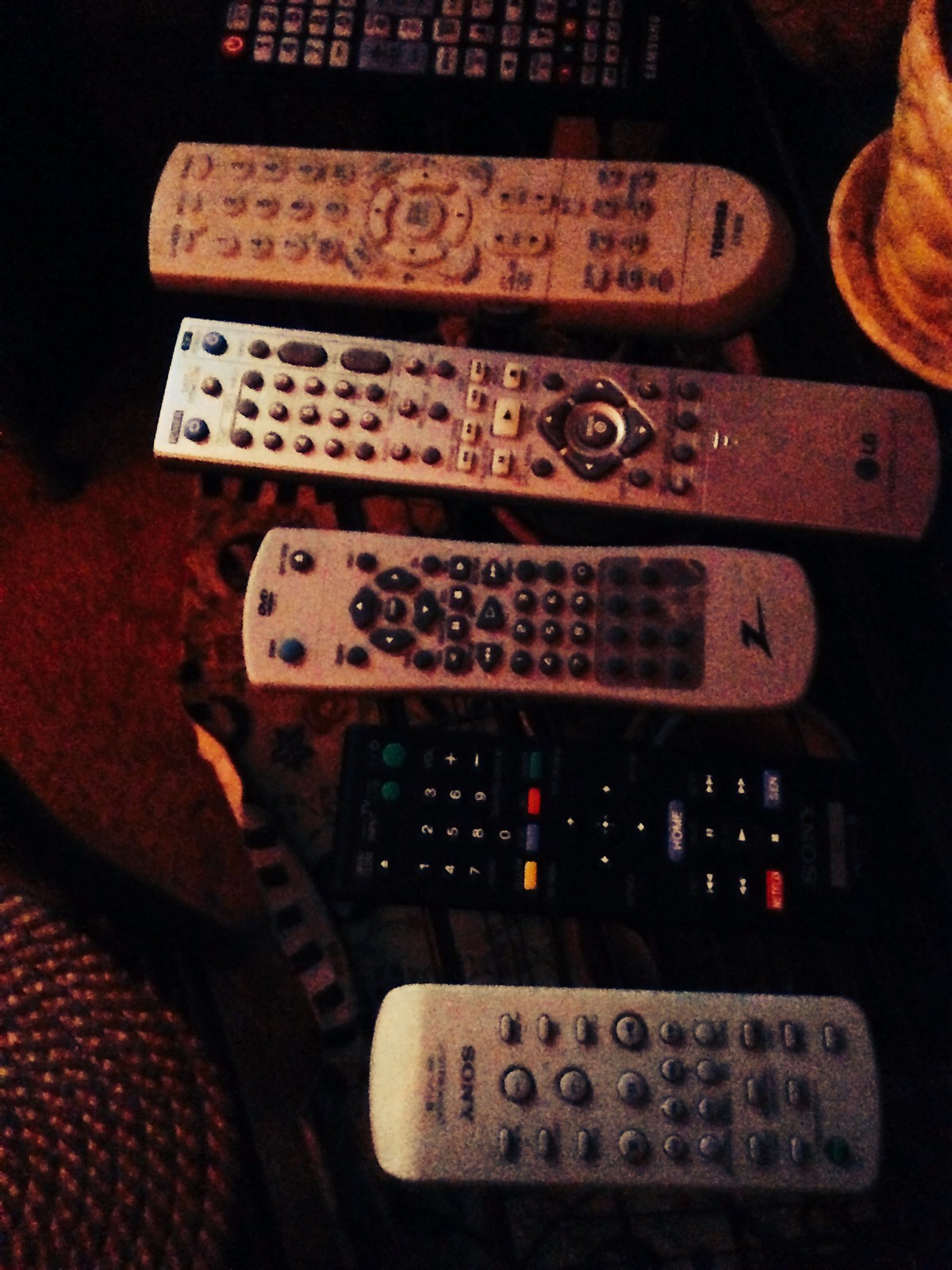This image depicts six remote controls of various sizes and colors, arranged from largest to smallest in a vertical orientation. At the top is a black remote with numerous white buttons and a distinctive red power button. Below it is a whitish Toshiba remote with white buttons marked by small black symbols. The middle features a prominent, long silver LG remote adorned with gray, white, and blue buttons. Next is another white remote bearing a little Z logo, likely for a DVD player, with contrasting black buttons. Following this, there is a black remote with a variety of colored buttons including yellow, blue, red, and green. The smallest remote at the bottom is a white Sony device with gray buttons. These remotes are placed on what appears to be a cluttered glass table with various background items such as rope placemats, leopard print paper, and potentially a coffee mug. The picture quality is somewhat grainy, giving it an old-school appearance.